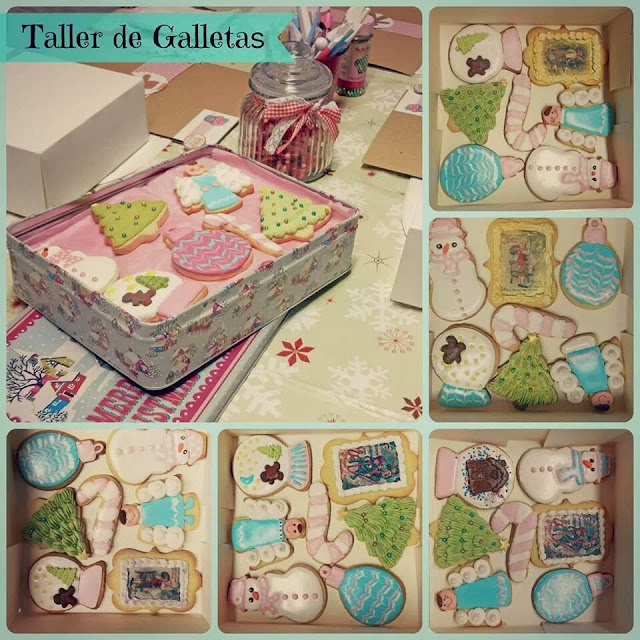The image is a collage set against a teal background, composed of one large square image in the upper left corner and five smaller squares arranged to the right and below the main picture, forming a larger square altogether. The main picture prominently features the title "Taller de Galletas" in black letters atop a teal banner. It showcases a festive assortment of colorfully decorated Christmas cookies, including shapes like a Christmas tree, an angel, an ornament, a snowman, and a candy cane. These cookies are neatly arranged inside a patterned gray cookie tin lined with pink paper, placed on a cheerful, festive tablecloth. Surrounding the tin, the background reveals additional holiday-themed items like glass containers holding pens and a white bakery box.

Each of the five smaller images offers slightly varied overhead views of the cookies, highlighting different angles and arrangements. Notably, these smaller images capture intricate details such as a snowman with a pink scarf and hat, an angel with white marshmallow wings, and candies like a lollipop with a pink stem. Across these images, consistent elements like Christmas trees with various colored dots, a white disc with a green Christmas tree, and differently styled snow globes are seen, emphasizing the festive theme. This collage likely represents a company specializing in holiday cookies, intending to showcase the variety and intricate designs of each cookie.